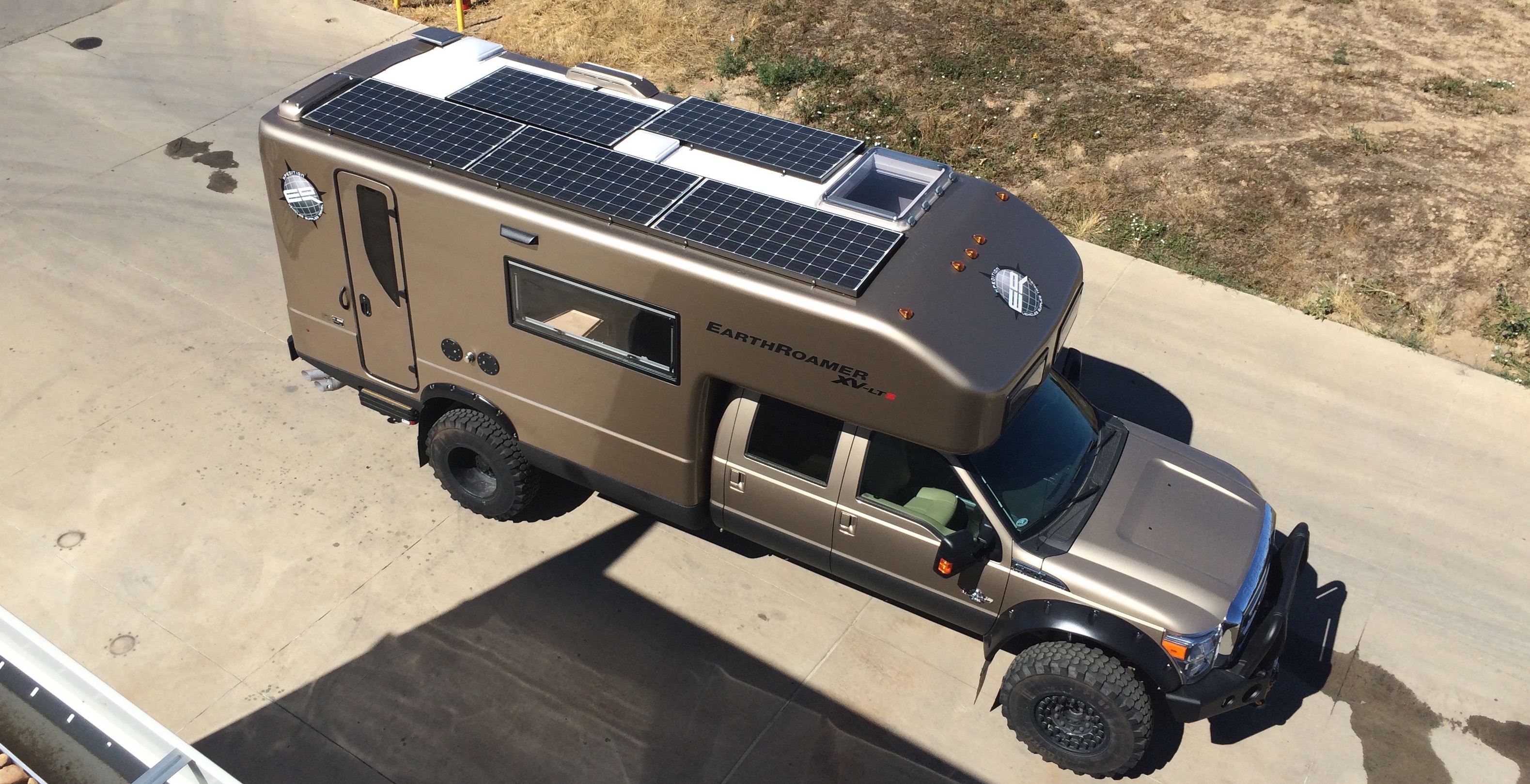An aerial shot, possibly from a taller building or helicopter, captures a rugged outdoor scene. A heavy-duty truck and an attached RV camper are parked on a dusty, desert road, bordered by patches of dead, brown grass and sparse green vegetation. The vehicle, painted in a metallic bronze or light brass color, contrasts sharply with the light limestone-colored road. The truck boasts large, impressive wheels and an aggressive front bumper with substantial grates around the headlights. The attached trailer, labeled with "Earth Roamer XV" in bold black letters, features five solar panels on its roof, suggesting a self-sufficient, mobile lifestyle. The overall composition highlights the vehicle's robust build designed for off-road adventure.